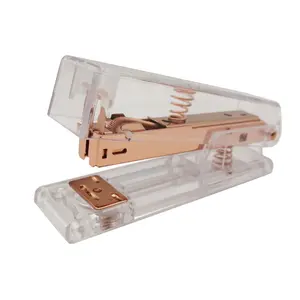This image showcases a translucent stapler placed against a white background. The clear plastic casing reveals the intricate metal internal parts and springs within. The stapler's design includes a large spring on the top side and another on the base, both visible through the clear plastic. The internal components and the base, where the stapling mechanism compresses the staple, are not see-through and feature a light copper, almost pinkish finish. The stapler is oriented with the working end on the left, angled slightly towards the viewer. There is no paper present in the image. The overall color palette includes whitish-gray translucent parts and light to dark brown metallic elements.